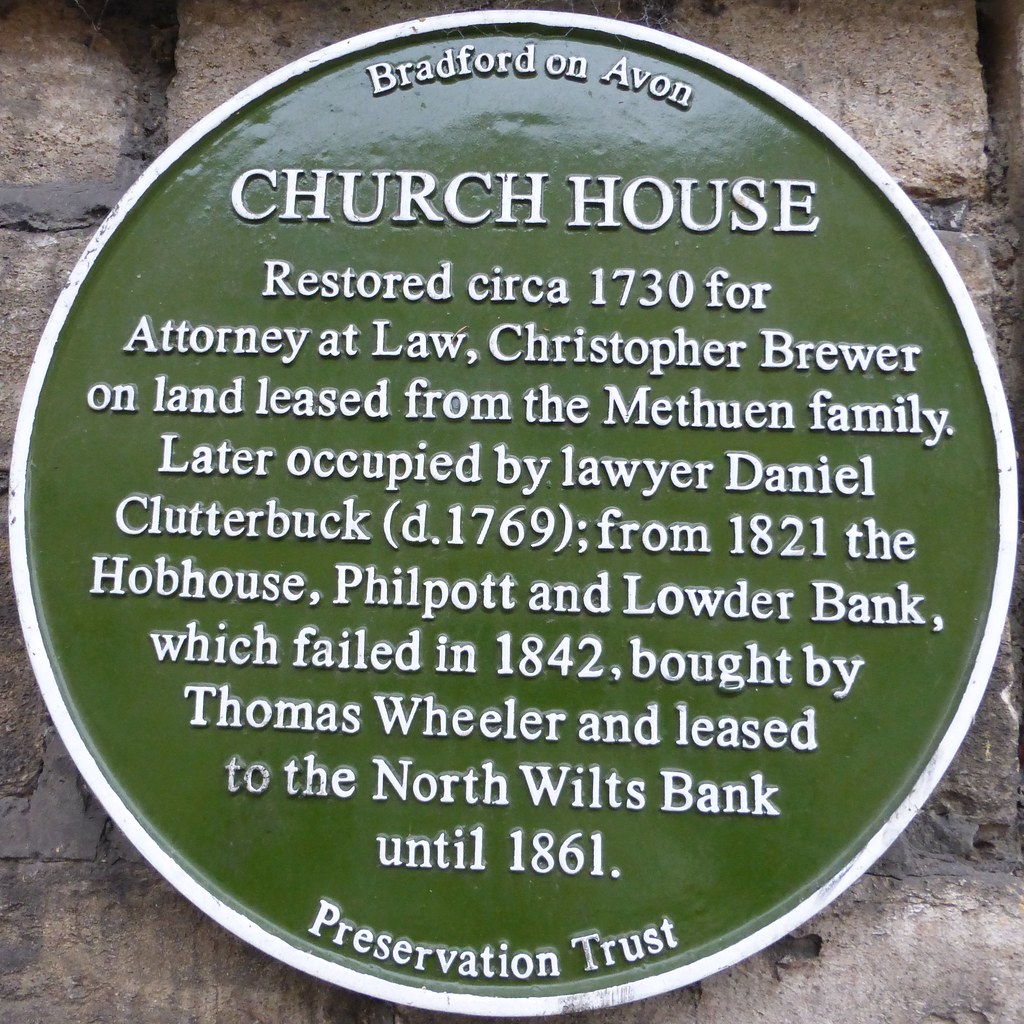This image features a circular green plaque with a silver border, mounted on a gray stone wall. The plaque, adorned with white text, has a shiny finish that reflects the light. At the top, it reads "Bradford on Avon," and following the border in big letters it says "Church House." The inscription narrates the history of the building: it was restored around 1730 for attorney-at-law Christopher Brewer on land leased from the Methuen family. The plaque details subsequent ownership, noting that lawyer Daniel Clutterbuck, who died in 1769, later occupied the house. From 1821, it became the Hob House associated with Peel, Fox, and Louder Bank, which failed in 1842. Thomas Wheeler then purchased it, leasing it to the North Wilts Bank until 1861. The marker concludes with a mention of the Preservation Trust. The detailed history encapsulates the building's long and varied past.